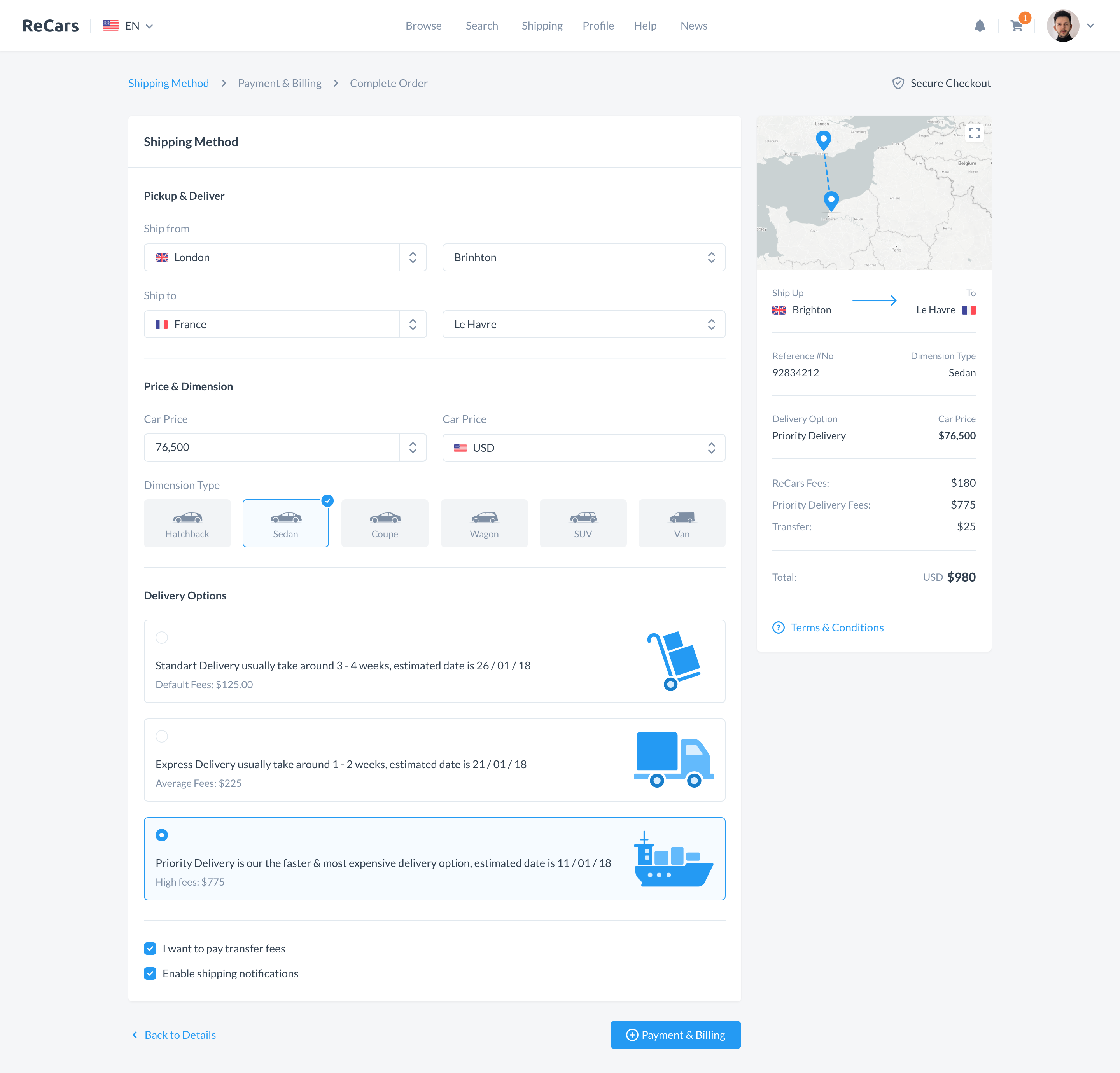This image shows a detailed interface of the ReCars website, specialized in car deliveries and purchases. The webpage visible is a form detailing the various stages of completing an order: Shipping Method, Payment and Billing, and Complete Order. The Shipping Method section highlights options like "Pick Up and Deliver," allowing cars to be shipped across Europe with accompanying fee details based on vehicle type—whether a hatchback, sedan, or coupe. Users can opt to pay transfer fees and enable shipping notifications. 

At the top, the site features a navigation menu with options for browsing, searching, shipping details, user profiles, help, and news. On the right side, there's a summary of the user's account, notifications, and cart contents, potentially containing a car. Despite appearing like a mockup, the caption confirms the website is genuine, as verified through a direct visit to the actual ReCars site.